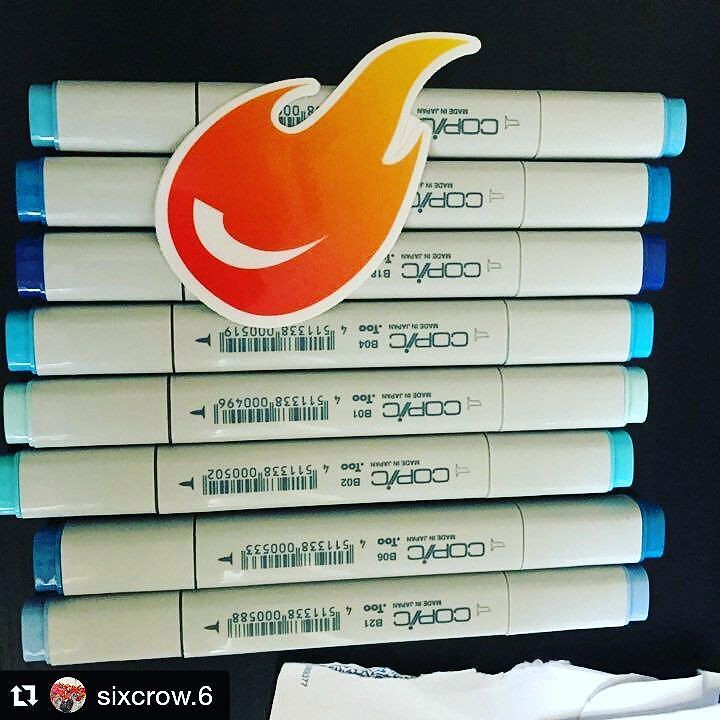The image showcases eight horizontally stacked Copic brand alcohol markers, each featuring a different shade of blue, displayed against a black table in a top-down perspective. The markers themselves are white with their tips showing various tones of blue, and the text on them is upside down to the viewer. Among the markers, there is a vibrant sticker depicting a stylized flame with a gradient transitioning from red at the base to yellow at the tip, accented by a white swoosh. In the lower left corner, a black rectangle houses two squared arrows forming a recycling-like symbol, accompanied by white text that reads "SixCrow.6." The background also includes a small image, potentially of red flowers in a black pot, although the details are difficult to discern. Additionally, a torn envelope rests in the bottom right corner of the image. The arrangement of the markers appears random concerning their shade, with the lightest and darkest shades not following any particular order.